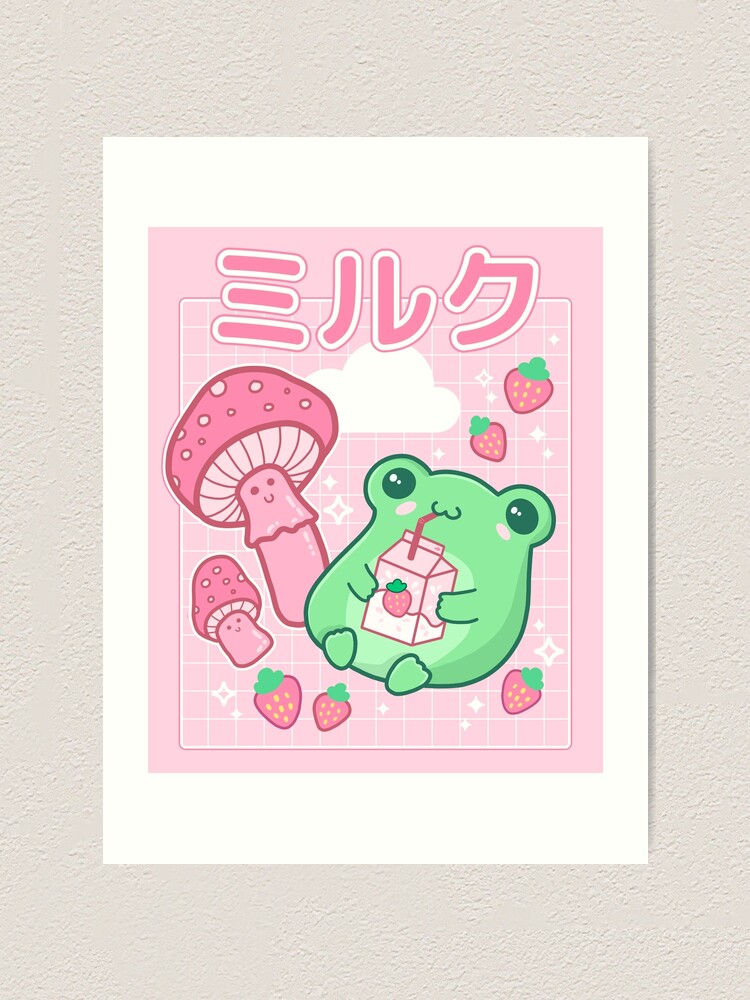This image is a digital color illustration in portrait orientation, mounted on a light beige wall. The artwork is framed with a white border, emphasizing its unique, kawaii Japanese style. The background of the art features a light pink rectangle with a soft white grid pattern overlay. At the top of the illustration, three dark pink Japanese kanji characters, outlined in white, are prominently displayed, adding an authentic touch. 

On the left side of the image, two cheerful, pink-capped mushrooms with smiling faces contribute to the whimsical atmosphere. The central figure is an adorable, lime green frog, often referred to as a cottagecore frog, lying back with its belly up, sipping from a small juice carton that has a red straw and a strawberry emblem. Surrounding the frog are five floating strawberries, adding a pop of color, and twinkling stars along with white clouds emphasizing the dreamy quality of the scene. The harmonious blend of these elements makes the illustration both captivating and delightfully cute.